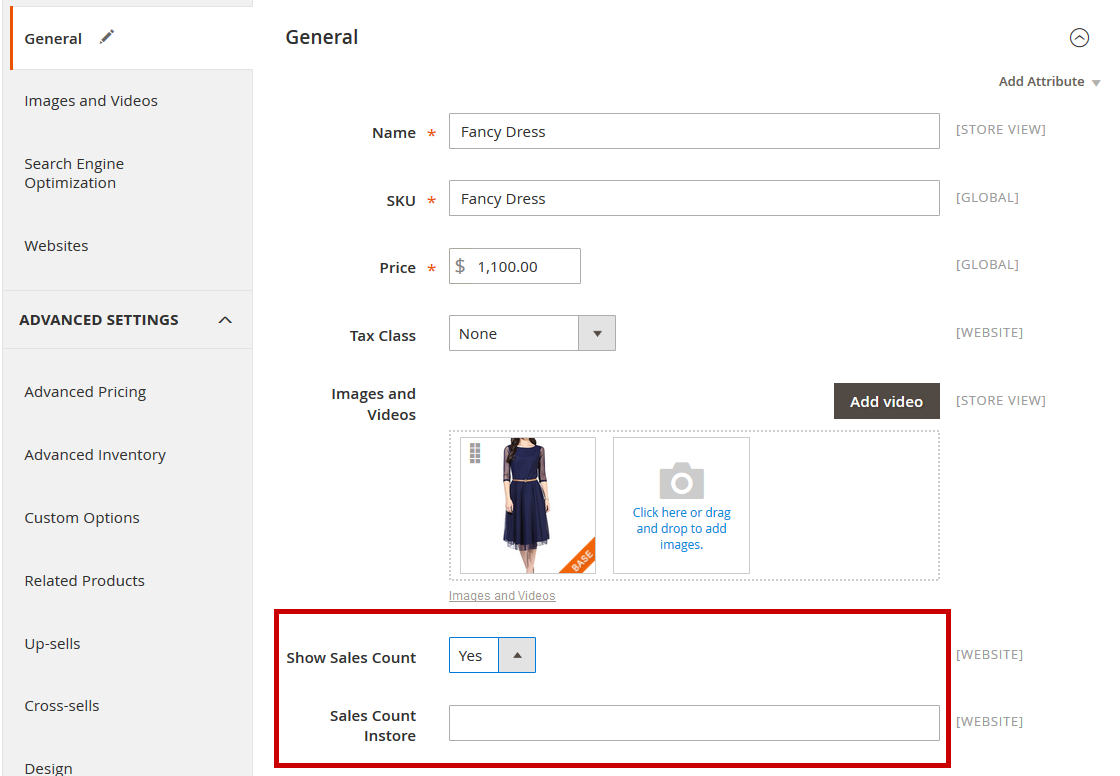On the left-hand side of the image, the interface is predominantly gray and black. The section titled "General" is highlighted in white, indicating that it is currently selected. Adjacent to this highlighted section, there is an orange-reddish line with a gray pen icon. Beneath this, various categories are listed in black text, including "Images," "Search Engine Optimization," "Websites," "Advanced Settings," "Advanced Pricing," "Advanced Inventory," "Custom Options," "Related Products," "Upsells," "Cross-sells," and "Design."

In the central white background area of the interface, the word "General" appears again in black. The form fields beneath it begin with "Name," followed by a mandatory red asterisk, and an input box where "Fancy Dress" has been typed in. Next, the "SKU" field also has a red asterisk, with "Fancy Dress" entered in the input box. The "Price" field features a similar input box with a gray dollar sign and the value "1,100.00." Following this, there is a "Tax Class" field displaying "None" in black text.

Accompanying this, an image or video section shows a female model wearing a navy blue dress, though her head is cropped out of the frame, leaving only her fair-skinned lower half visible. 

At the bottom of the interface, a red rectangular outline highlights a section labeled "Show Sales Count." It is marked with "Yes," indicating that sales information should be displayed. The "Sales Count in Store" is shown as an empty white rectangular input box, indicating that the actual number of sales has not yet been inputted.